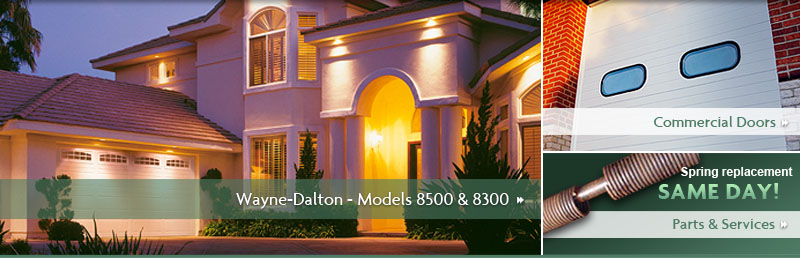This image appears to be a promotional banner typically found at the top of a website, advertising various garage door products and services from the company Wayne Dalton. The largest image on the left showcases the facade of a two-story house illuminated during dusk, with its porch lights and garage lights turned on, creating a warm and inviting ambiance. The garage door is clearly visible, and an opaque green stripe at the bottom of this image displays the text "Wayne Dalton models 8500 and 8300," along with a clickable forward arrow.

On the right side, there are two smaller, clickable images stacked vertically. The top image features a commercial roll-up garage door, with the text "Commercial Doors" indicating it can be clicked for more information. Below it, the bottom image highlights the services offered by the company, with text reading "Spring Replacement Same Day" and "Parts and Services." This image includes a visual of a garage door spring in the top left corner, suggesting the reliability and availability of their repair services.

The image lacks any navigational elements like taskbars, toolbars, login options, or contact information, indicating it is likely a cropped section from the website’s header, focusing solely on showcasing the products and services without additional site navigation or branding details.